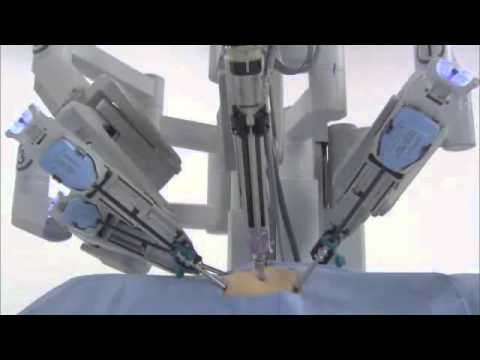The image depicts a hospital setting where a sophisticated robotic surgical apparatus operates. The scene shows a blue surgical drape with a hole revealing skin in the center, suggesting the patient is prepped for surgery. The machine features five mechanistic arms equipped with various medical instruments, including needles, syringes, forceps, or clamps, and hoses for maneuvering the arms. The surgical table, also blue, appears to support the patient, with the drape covering most of their body. The skin within the hole remains uncut, indicating the procedure is about to begin, conducted entirely by the robotic system without direct human intervention.